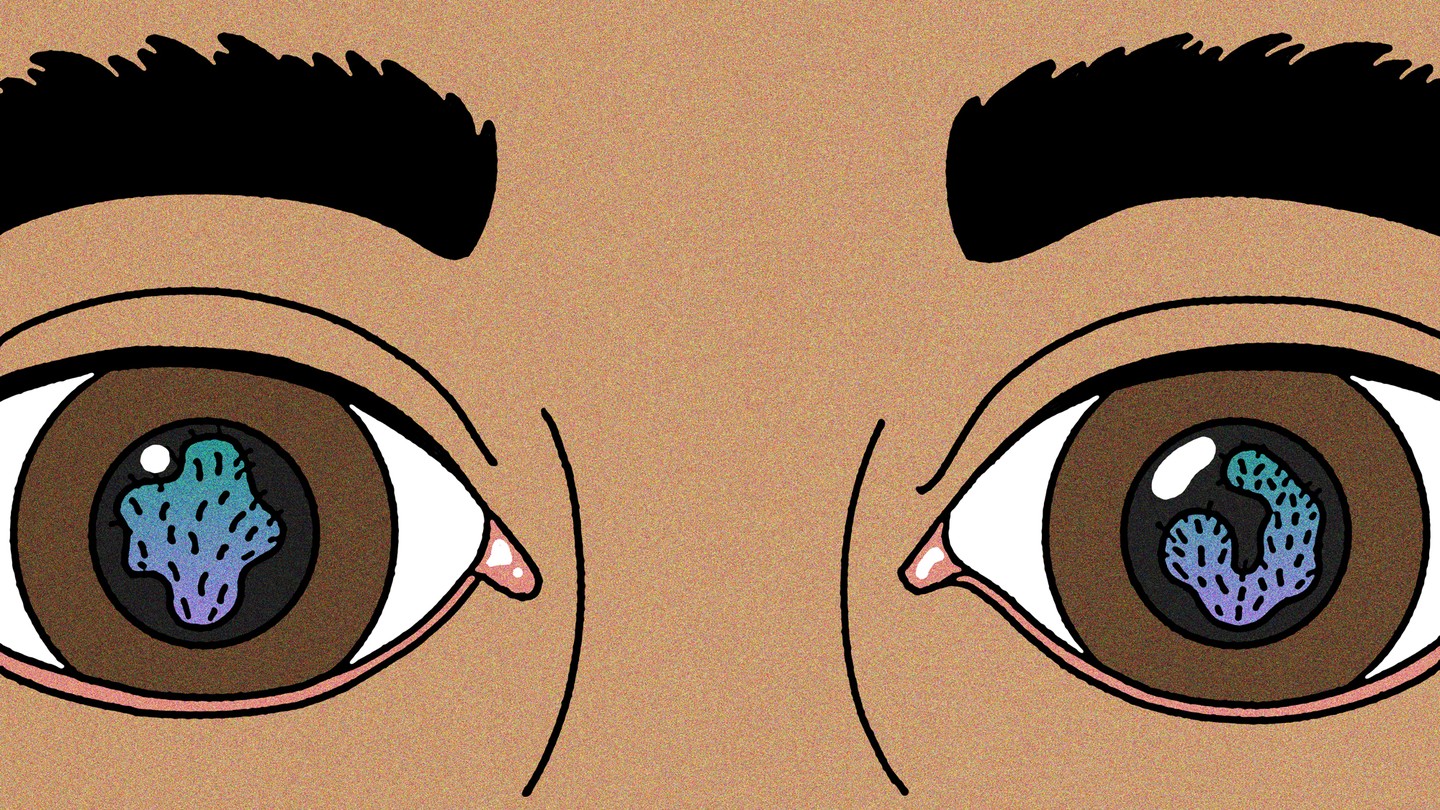This is a detailed computer-generated cartoon drawing, presented in a horizontal rectangular frame, focusing closely on a person's eyes, eyebrows, and surrounding skin. The person depicted has light brown skin indicative of a black individual, and bushy, dark black eyebrows. Central to the image are the person's dark brown eyes, each featuring unique and intricate details within the irises. The left eye contains a green and purple splotch resembling an amoeba, accentuated with black lines and a tiny white circle above it to the left. Similarly, the right eye displays a backwards C-shaped splotch of the same green and purple color, with a small white oblong shape located above it. The drawing utilizes brown skin tones and emphasizes the emotional depth in the character's eyes, possibly suggesting the onset of tears. The style of the illustration resembles that of characters from the TV cartoon show "The Bone Docs."